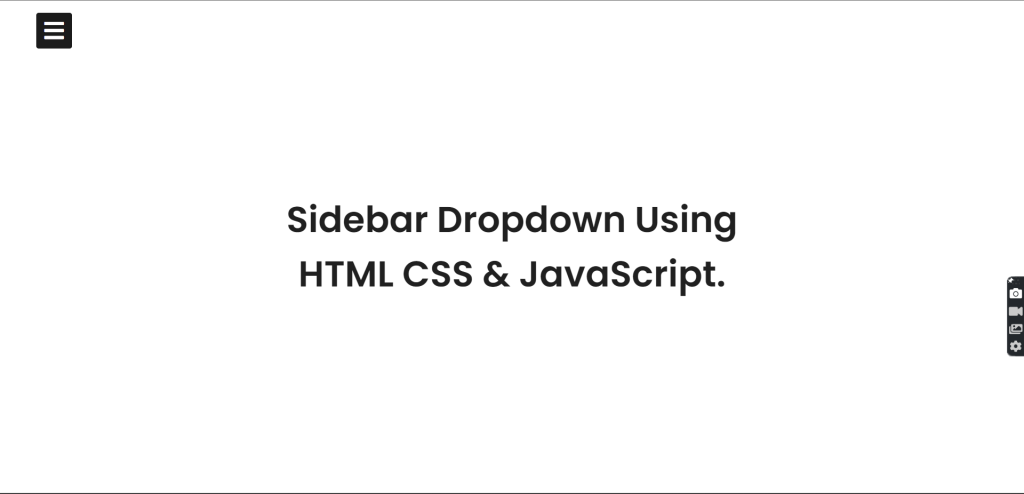The image is a horizontally rectangular screenshot set against a white background. In the upper left corner, there is a small black box featuring three horizontal bars, representing a menu icon. Dominating the right side of the image, just below the center, is a narrow, short, vertically aligned black strip housing four distinct icons: a camera, a video camera, a picture-in-picture symbol, and a settings icon, stacked from top to bottom. The focal point of the image is centrally placed text, presented in bold black font across two lines. The first line reads "sidebar drop down using," while the second line states "html, css, and javascript." The sparse nature of elements within the image suggests that it is likely a screenshot.